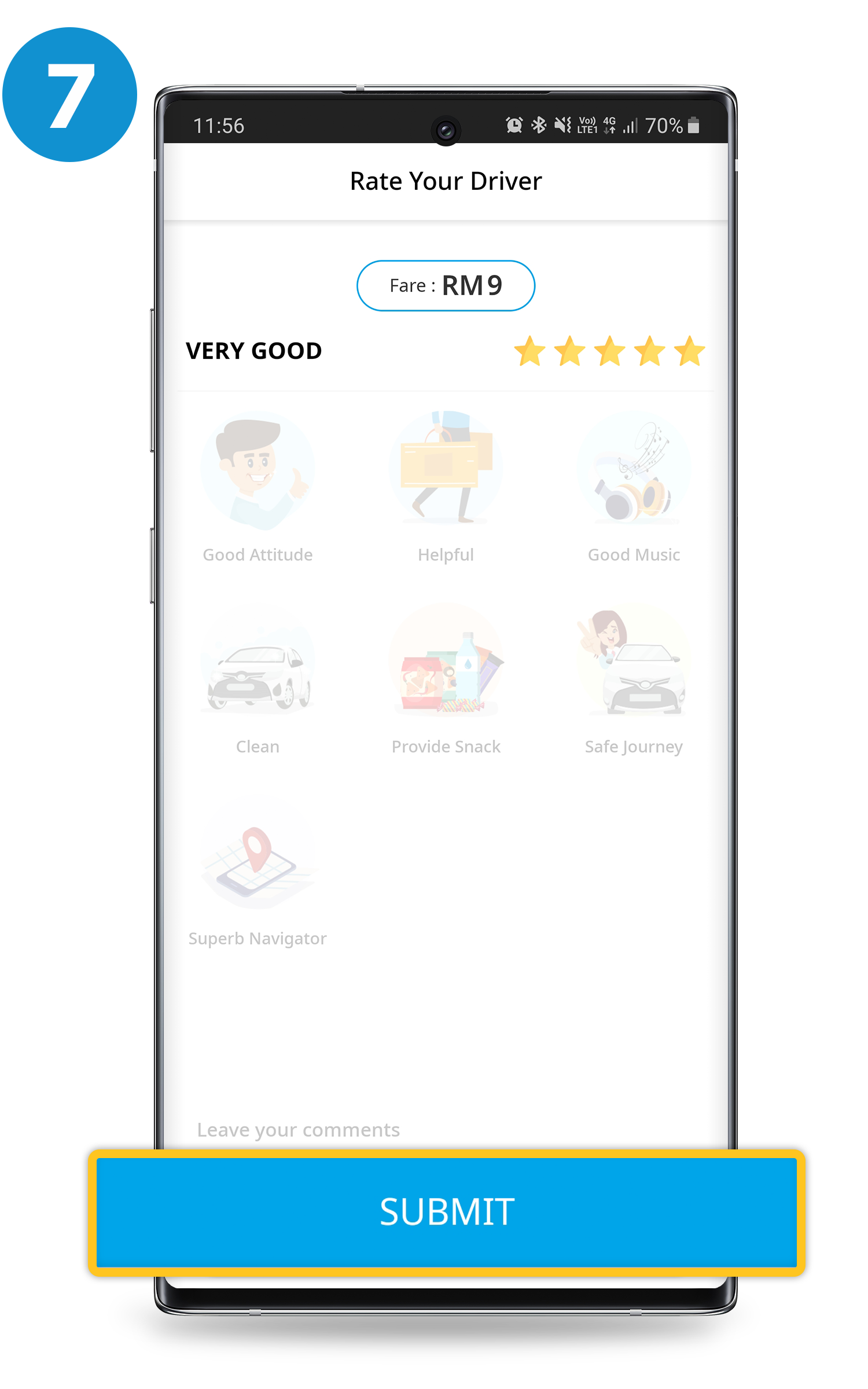This image features a modern cell phone prominently displayed against a white background. The cell phone has visible buttons on its side, and its screen is active. In the top left corner of the white background, there is a blue circle with a white number "7" inside, suggesting some instructional context.

The cell phone’s display shows detailed information:
- **Top bar details:** The time is displayed as 11:56. Next to it are icons indicating an active alarm, Wi-Fi connectivity, and that the phone is in vibrate mode. The screen also shows 4G signal strength with four bars and a 70% battery level.
- **Middle of the screen:** The name "Rachel Driver" is prominently displayed.
- **Below the name:** A gray dividing line separates the name from the fare information, listed as "Fare: RM9". 
- **Rating information:** It shows a rating of "Very Good" along with five stars.
- **Additional details:** There are numerous icons below the mentioned ratings indicating qualities such as a good attitude, helpfulness, good music, cleanliness (provided snacks), a safe journey, and superb navigation skills.

At the bottom of the phone screen, a message invites users to "leave your comments". Overlaying the phone’s screen is a "Submit" button, which is blue with a yellow outline, suggesting this is an interactive feature for submitting feedback.

The entire image is accented with colors such as blue, white, black, gray, and yellow, and seems to be part of a step-by-step instructional guide, possibly indicating this is step number seven in a series.